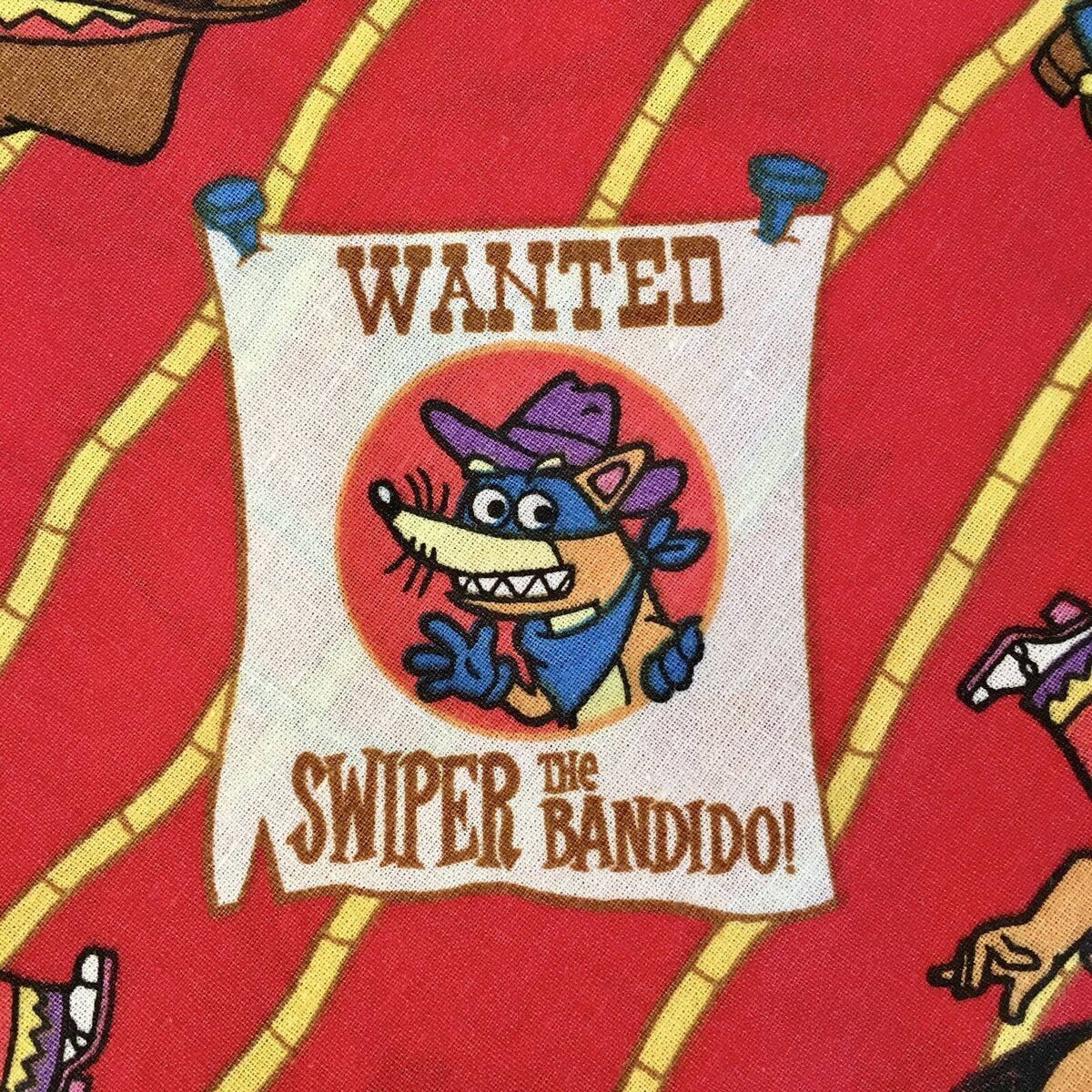The image showcases a close-up of children's pajamas, specifically focusing on a cartoon illustration inspired by a wanted poster. The fabric is predominantly red with yellow, bamboo-like diagonal stripes. Central to the image is a large square with a red background intersected by yellow lines resembling ropes. Within this square is a white section featuring a playful wanted poster that reads, "Wanted, Swiper the Bandito." The poster includes a circular portrait of Swiper the Fox from Dora the Explorer, depicted as an old western bandit. Swiper has an orange and yellow coat, a purple cowboy hat, a blue bandana, blue gloves, a black eye mask, and a white snout with black whiskers. The poster is pinned at the top with two metal pins. Surrounding this focal point, though partially off-screen, are elements of other characters and designs, including a glimpse of Dora’s arm.